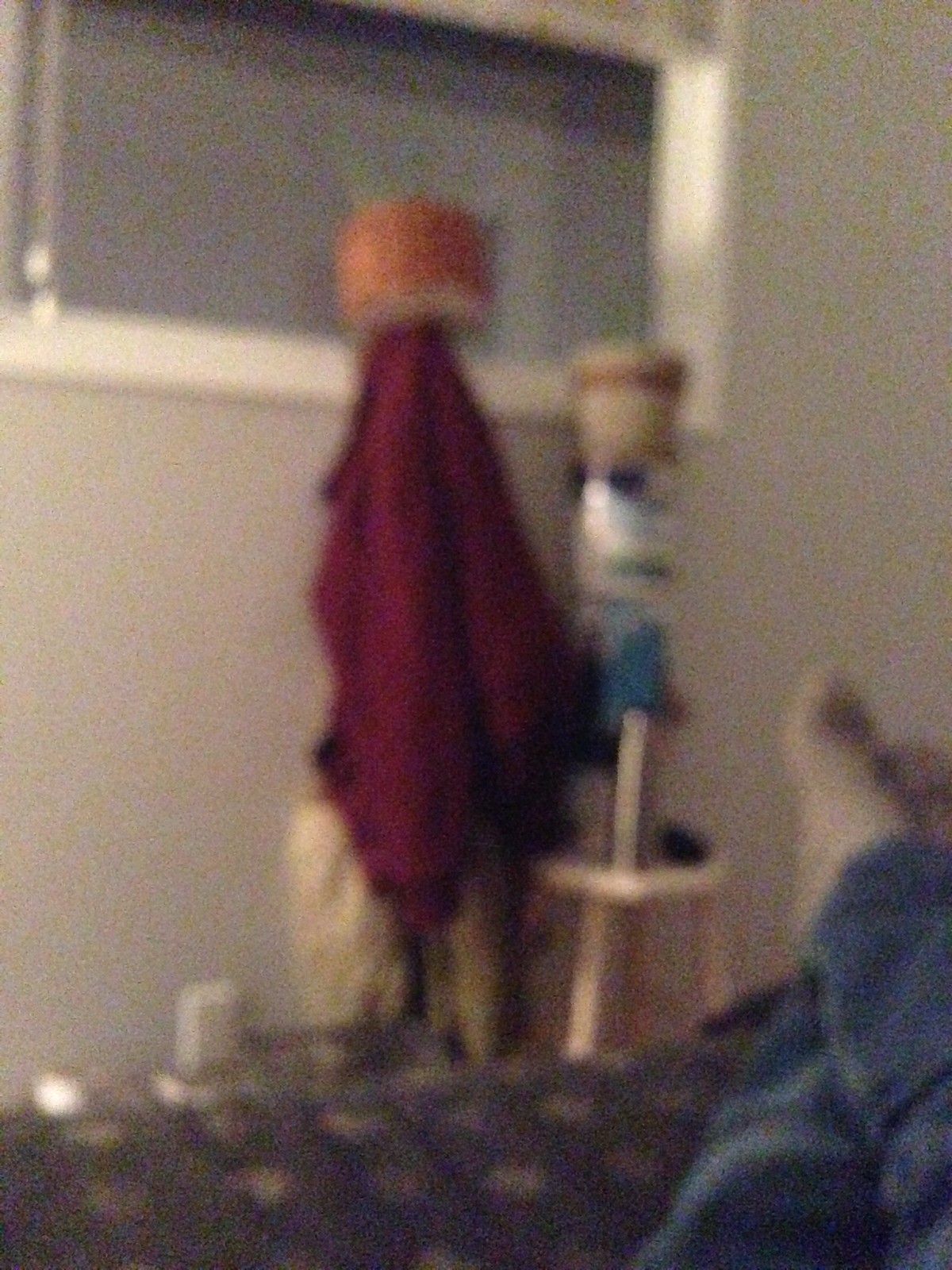This photograph captures a moment of relaxation as viewed from the perspective of someone lying in bed. Despite the grainy quality of the image, certain details stand out. The individual is dressed in light blue jeans and white socks, with their legs comfortably crossed right over left. They are resting on a bed adorned with a dark blue comforter featuring white polka dots. The focus of the photograph appears to be directed toward a white wall. 

In front of this wall, two coat hangers are positioned. The hanger on the right side is white and topped with a tan pot accented by a brown stripe. The hanger on the left side is distinguished by a brown cylindrical object resting on its top. Beneath this, a dark red, long-sleeve jacket is draped, accompanied by a tan-colored jacket hanging underneath. The assortment of personal items and the casual composition provide a glimpse into a cozy, intimate space captured in an unguarded moment.